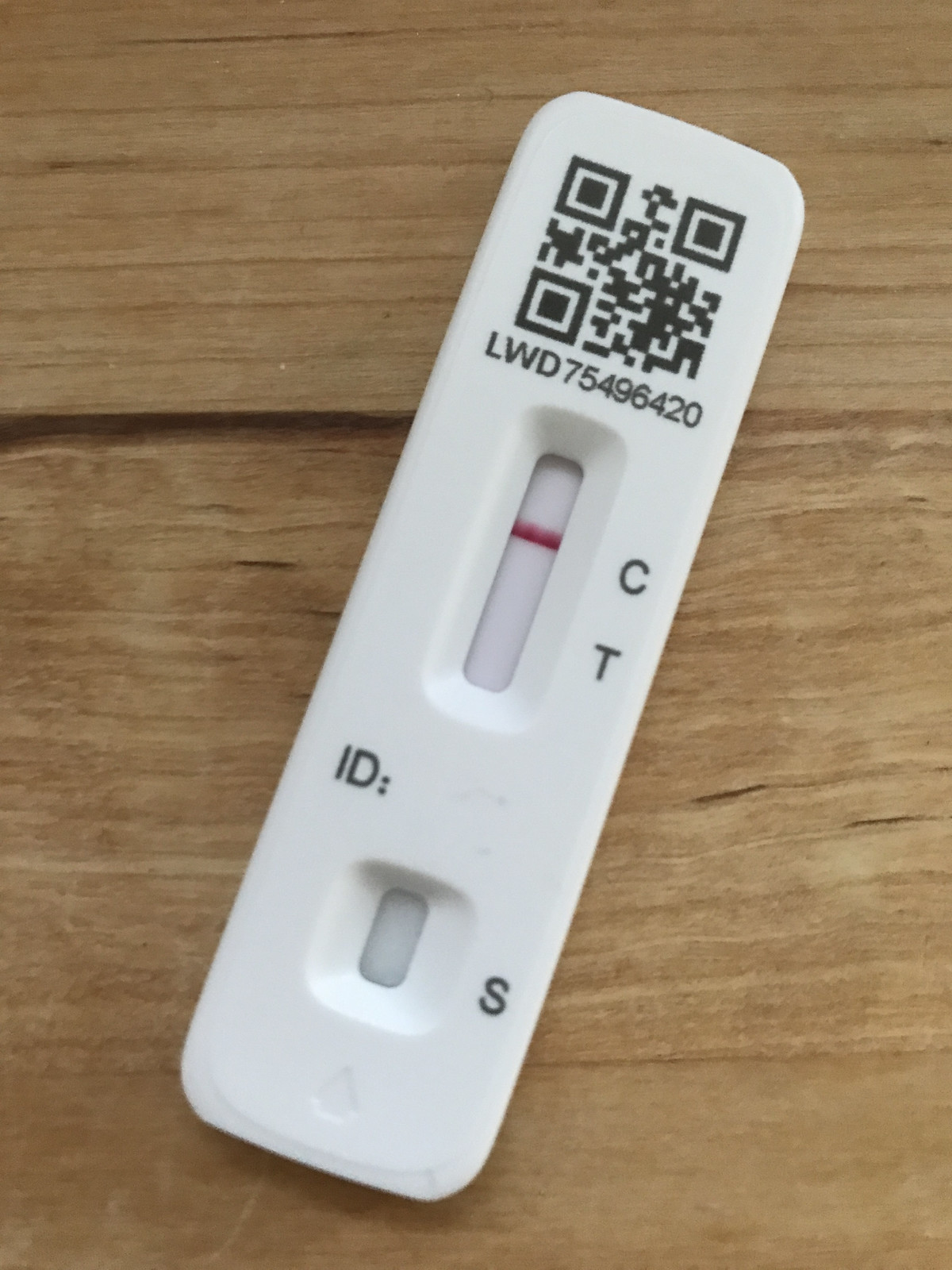This detailed photograph captures a white rapid test resting on a dark brown wooden surface with visible wood grain. The test, predominantly black and white, features a QR code in black at the top, followed by an alphanumeric string. In the center of the test, there's a white notch with a prominent red line next to the letter 'C' in black font. Below the red line, towards the bottom of the test, there is another white notch labeled 'ID' in black. Furthermore, there is a small black 'S' visible near a teardrop-shaped cutout at the bottom of the test strip. The image is crystal clear, with no additional objects present, emphasizing the contrast between the white test and the dark wooden table. A portion of the table exhibits a lighter, almost white appearance, adding to the visual elements of the photograph.